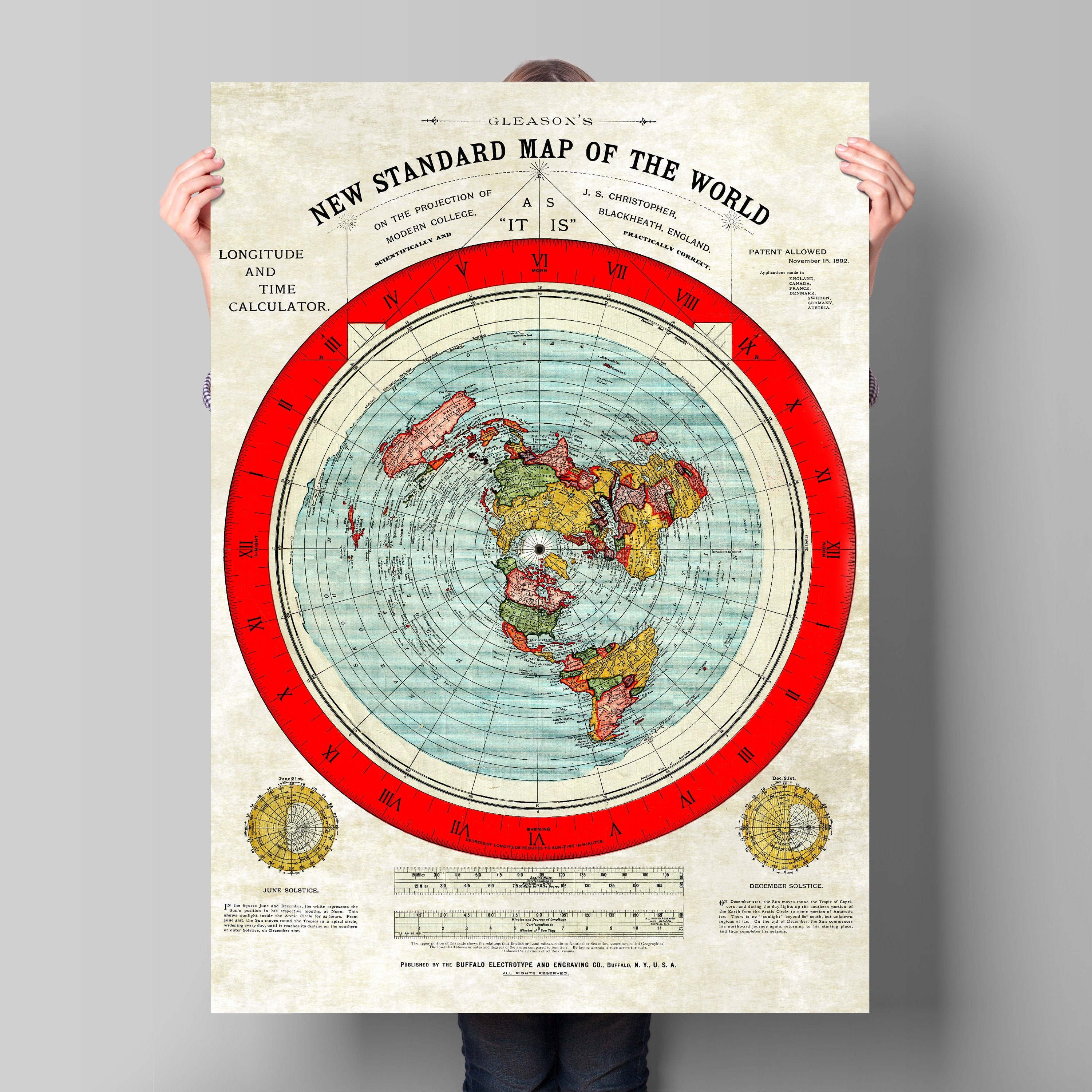In the image, a person with blonde hair is holding a large, detailed map titled "Gleason's New Standard Map of the World." The person is standing in front of a gray wall, with only the top of their head, their hands, and a small portion of their jeans visible around the edges of the poster. Their hands grip the top corners of the map, with the back of their fingers showing. The map itself is primarily gray and features a central circular depiction of the globe, surrounded by markings and text. A red trim with Roman numerals encircles the map. Just below the person's head, the title "Gleason's New Standard Map of the World" is printed in bold letters, with smaller, unreadable text beneath it. The poster also includes a section at the bottom that appears to be a table of contents. In the bottom corners of the map are gold circles with indecipherable markings. Additionally, the map contains the phrases "Longitude and Time Calculator" and "On the Projection of Modern College," alongside references to the December solstice and June solstice. The map reaches almost from the top to the bottom of the image, leaving only an inch or so of the background visible on either side.